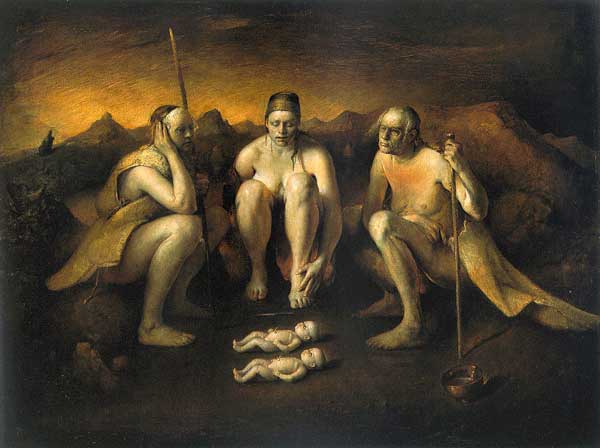This painting depicts a somber scene of three women arranged in a semi-circle around two nearly identical, pale infants lying on the ground. The overall color palette is dominated by browns, yellows, and shades of gold, lending the image a sepia-toned, melancholic atmosphere. In the background, a dismal sky fades from dark brown to a golden orange near the horizon, possibly hinting at a setting or rising sun.

The woman on the left is seated on rocks, dressed in a yellow robe, and holding a staff or stick. Her right hand is covering her ear, adding to the sense of sorrow that pervades the scene. The central woman faces the viewer directly, with her knees drawn up to her chest; she appears to be the youngest of the three and is quite possibly unclothed. The woman on the right, who seems to be the oldest, also holds a staff and is crouching down.

Both infants lie side by side between the women, their heads oriented to the right. They, like the women, are very pale, almost ghostly. On the ground to the right of the infants, there is a small, bronze-colored bowl, adding a mundane touch to the otherwise haunting tableau. The backdrop includes distant mountains, contributing to the image's forlorn and eerie mood.